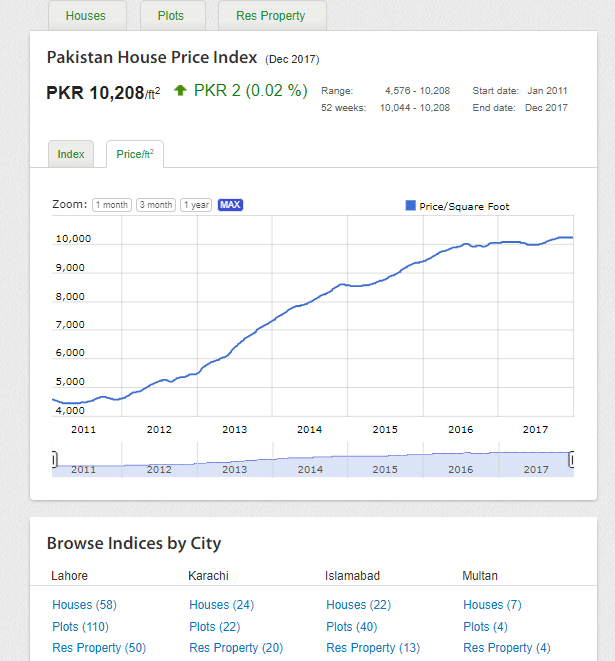This detailed chart presents the Pakistan House Price Index as of December 2017. The graph delineates the performance and trends in residential property prices over the past six to seven years. 

At the top, three headers are prominently displayed in green letters set against a gray background. The body of the chart features data in white, clearly marked with categories: "Houses", "Plots", and "Res. Property". Beneath these categories, the index is labeled as the "Pakistan House Price Index, December 2017" with the index symbol "PKR". The chart specifies a value of 10,208 PKR per square foot and notes a marginal increase of PKR 2, representing a 0.02% rise. The 52-week range for the index is documented as 4,570 to 10,208 PKR.

The vertical axis on the left side of the chart is scaled from 4,000 to 10,000 in increments of 1,000, facilitating a visual representation of price trends. The horizontal axis at the bottom charts the years from 2011 through to 2017, showing a steady increase in property values from 4,576 PKR in January 2011 to 10,208 PKR by December 2017.

The bottom of the chart includes a detailed legend titled "Brown Indices by City", listing major urban centers: Lahore, Karachi, Islamabad, and Multan, with a focus on house, plot, and residential property types. 

The graphical plot highlights the considerable appreciation of property prices over the specified period, providing a comprehensive overview of the housing market's upward trajectory in Pakistan’s major cities.